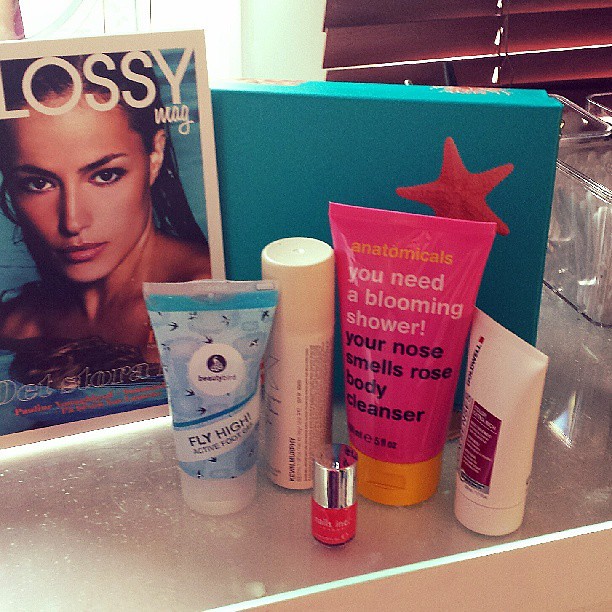This detailed close-up photographic image showcases a variety of beauty and personal care products arranged on a glass shelf, set against an interior backdrop that suggests either a home or a department store. Starting from the left, there's a tube labeled "Fly High Active Foot Cream." Beside it stands a small clear glass bottle containing red nail polish, topped with a silver cap. Moving right, there's a pink cylindrical tube, its ingredients listed but too fine to discern, and partially turned to obscure its label. Next is another tube labeled "Anatomicals: you need a blooming shower, your nose smells rose, body cleanser," measuring 5.9 ounces.

To the right of the cleanser, there is a beige tube with purple lettering, but the text is too small and the angle too poor to read. Behind these products, a vibrant blue box adorned with a starfish sits prominently. Over to the left in the background, a magazine cover titled "Glossy Meg" displays a young brunette woman immersed in water, gazing directly at the camera. This entire scene is softly lit by light filtering through brown venetian blinds and a nearby window.